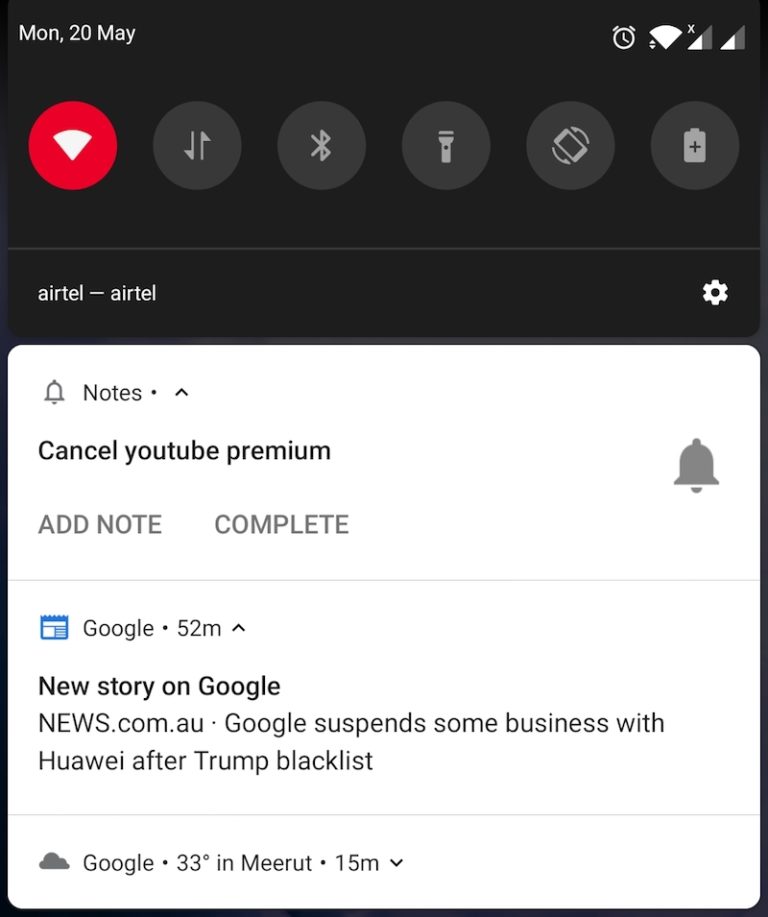In this image, we see a screenshot set against a black background. At the top, the text reads "Monday, 20th May" in white. In the upper right corner are icons for an alarm clock and Wi-Fi. Just below these, from left to right, is a red circle with a triangle inside it, which likely indicates a recording notification. Next to it are icons for a flashlight and battery status, followed by the "Airtel" network indicator. To the right of the network indicator is a white settings icon.

Below these elements, there is a rectangular white box with a slight black border on the right, left, and bottom. In the upper left corner of the white box are icons and text for notifications - first, a notification bell, and then the word "notes." Beneath that is the text "Cancel YouTube Premium," with a gray notification bell icon to its right.

Further down on the left side within the white box, there is an "Add note" option and a "Complete" button, separated by a thin gray horizontal line. At the bottom of the white box, there is a news notification from Google, reading: "52 minutes ago - New story on google.com.au: Google suspends some business with Huawei after Trump blacklist."